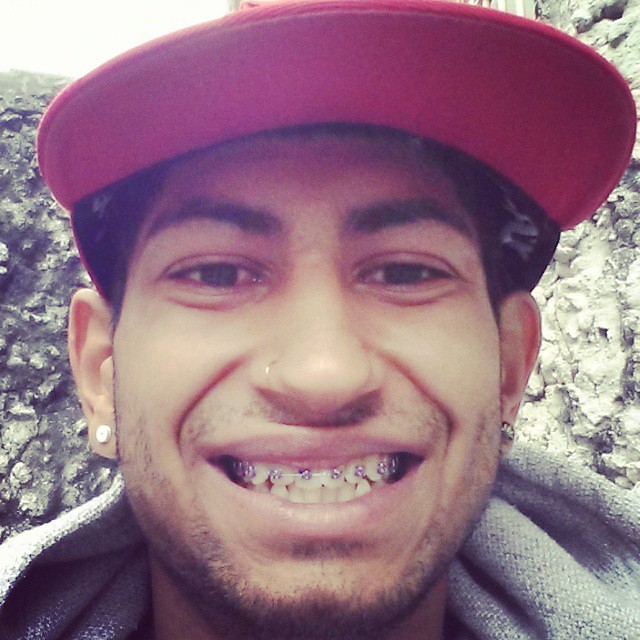This close-up photograph captures a man who appears to be Hispanic or Mediterranean, smiling broadly while showing off his silver braces, which are only on his upper teeth. He has a light, scruffy beard and short black hair, partially covered by his red baseball cap featuring a black underside. His facial accessories include diamond-like earrings in both ears and a nose ring in his right nostril. The man is dressed in a gray hoodie or a thick, coarse material shirt. The background is composed of rugged, jagged rocks in varying shades of gray and green, with a light source coming from the top left, suggesting an outdoor setting. The man’s happy expression and the very close framing of the shot imply it could be a selfie.